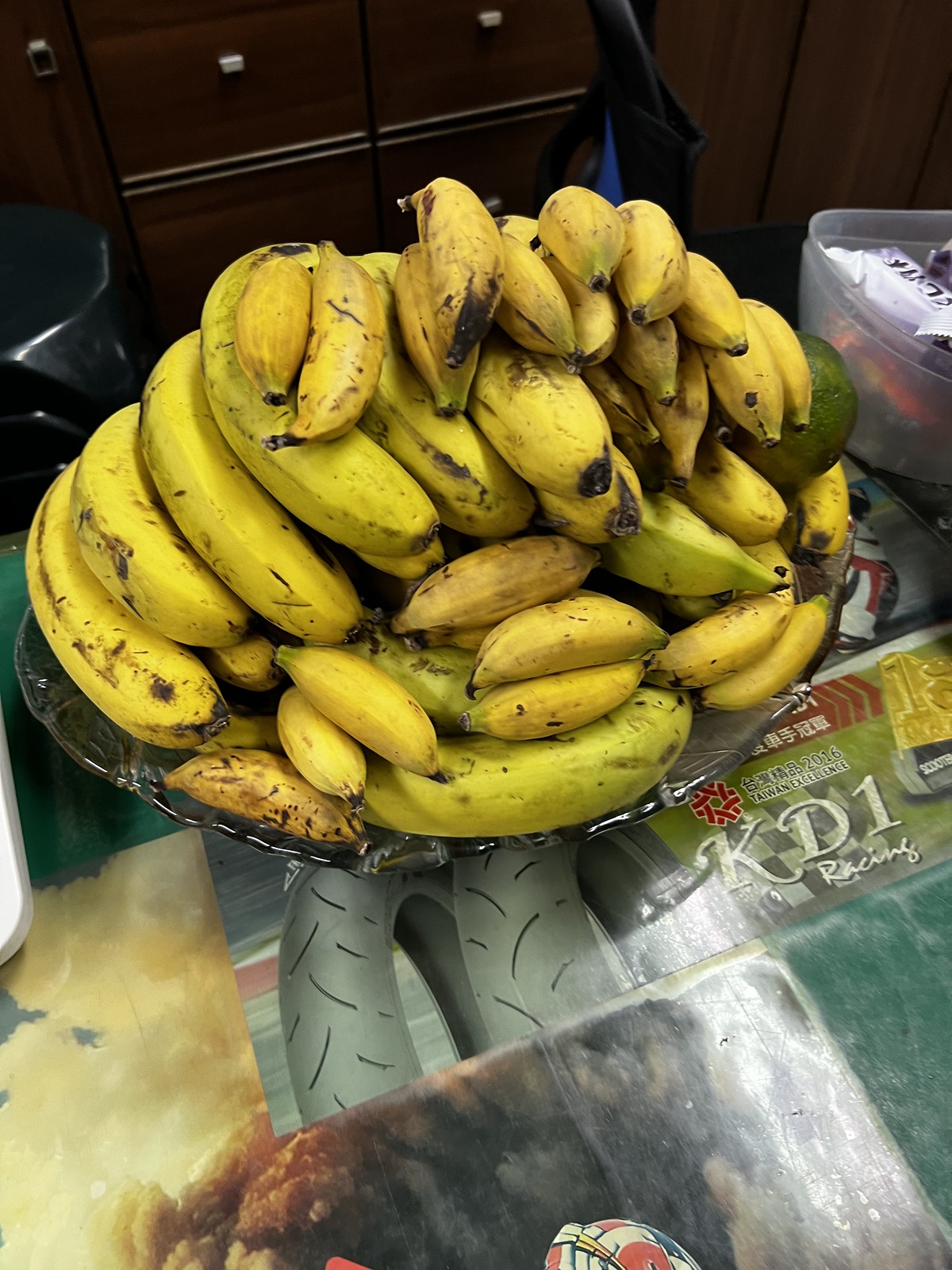The image is a colour photograph in a portrait orientation, with the main focus on a large stack of bananas and small plantains arranged on an oval glass platter that has slight undulations around its edge. The bananas are primarily yellow with green tinges and spots of brown and black, indicating they are beginning to ripen. The small plantains, mixed among the regular bananas, are a darker yellow. The glass platter underneath the fruit is mostly obscured by the abundance of bananas.

Beneath the platter, various graphical-type illustrations and photographic cards are partially visible. These include a grey tyre with black tread lines and some text reading "KD1 Racing" accompanied by Japanese characters. Other visible cards display a range of colors and designs, including one with green and brown hues and another potentially depicting a banana or corn. One card features a cloud-like pattern in yellow, and another has a partially visible letter that could be a "U" or an "O."

In the background, dark oak small drawers can be discerned, suggesting the image was taken in an indoor setting, though the exact location remains unclear. The varied colors and graphical elements beneath the platter, along with the ripe bananas on top, create a visually intriguing composition.